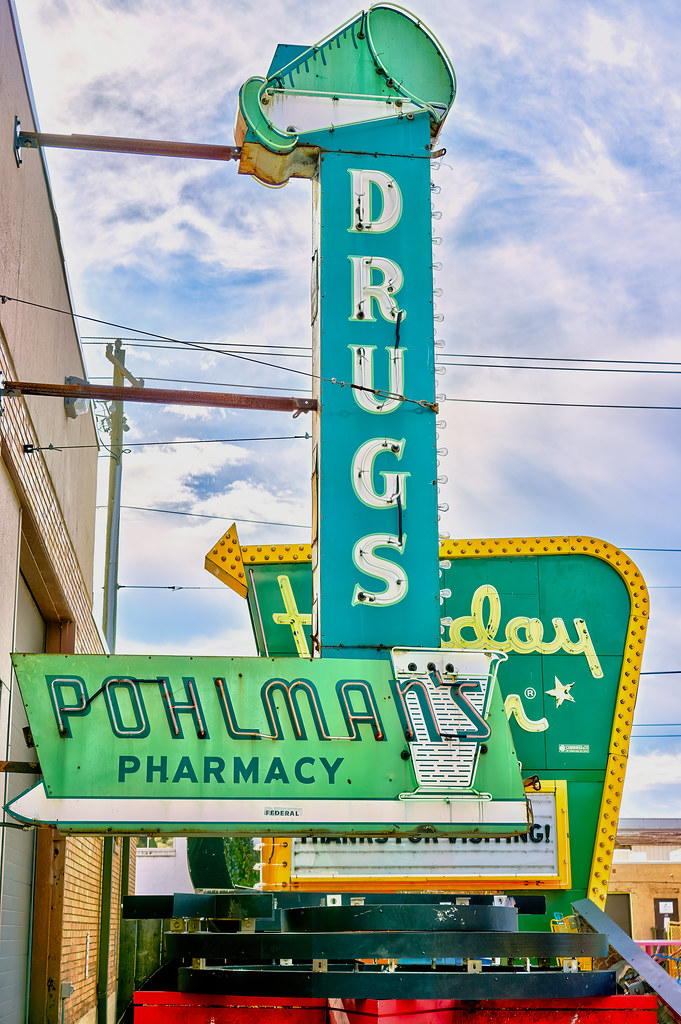The image depicts an outdoor scene next to a building, characterized by partly cloudy, wispy skies and a background of blue with feathery clouds. Prominently featured is a vertical sign with a light blue background and white lettering that spells out "DRUGS," topped with a green cylinder resembling a beaker with blue lines and white liquid inside, appearing as if it's being poured. The sign is affixed to what seems like a clay-like red or yellow brick building, upheld by two reddish, rusty poles.

Below the main "DRUGS" sign, there is another green-background sign that reads "Pullman's Pharmacy," though "Palms Pharmacy" is also mentioned, suggesting a possible variation or read error. The word "Palms" is outlined in yellow and green, with "Pharmacy" written in green on a similarly green background. 

To the rear of this setup, there's a "Holiday Inn" sign in yellow letters on a green background, highlighted with a yellow arrow pointing towards the building. The sign's precise content at the bottom is obscured, though there are hints of more textual information. 

Among the scene's additional elements are telephone poles, likely brown, with wires extending out of the picture frame, and assorted red and black metal objects, possibly large red totes with black bars resting on top. The exact details here are hard to discern as parts of the image are cut off. There's also a notable beaker-like design with blue or black lines on yet another sign, enhancing the pharmaceutical theme of the setting.